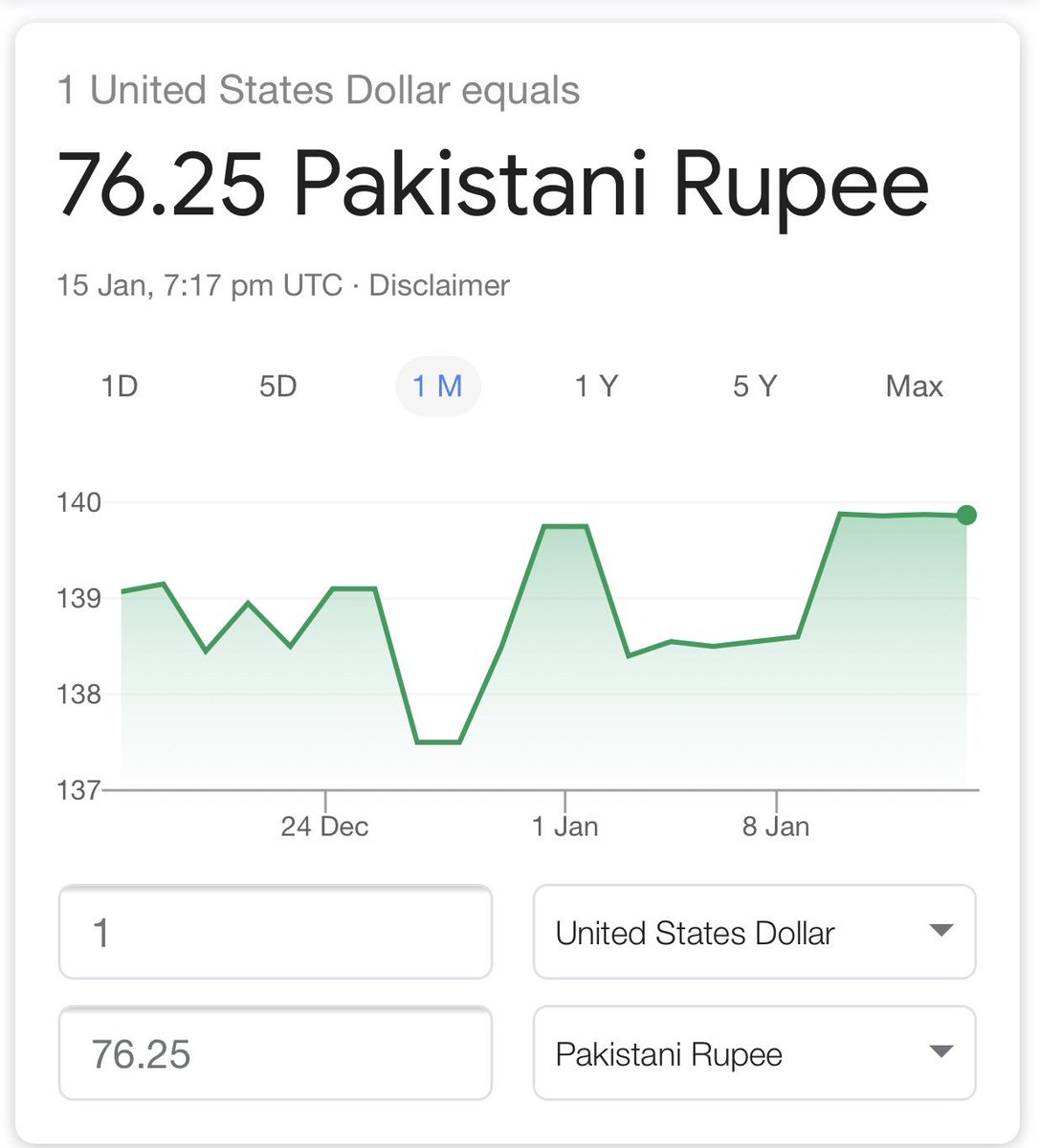The image displays a detailed financial graph on a screen with a white background, illustrating the exchange rate of the Pakistani Rupee (PKR) against the United States Dollar (USD). The graph is contained within a large, slightly taller-than-wide rectangle with a gray band at the top, where the text reads, "One United States dollar equals," followed by "76.25 Pakistani rupees" in bold black letters. Below it is a timestamp stating "15 January, 7:17 PM, UTC," along with a disclaimer.

At the top section below the title, there are six labeled buttons for selecting different time periods: "1D", "5D", "1M", "1Y", "5Y", and "Max". The "1M" (one month) option is selected, indicated by a gray circle around it and blue text.

The graph features a Y-axis ranging from 137 to 140 and an X-axis representing time, starting from "24 December" and progressing through "1 January" to "8 January". A green fluctuating line traces the exchange rate movement, starting slightly above 139, dipping to a low of approximately 137.5, and ending close to 140 by the end of the observed period.

Below the graph, there are four buttons for selecting different attributes. In the top row, the first button is labeled "1" (indicating the value of one unit) and "United States Dollar," which has a downward-facing caret, suggesting a dropdown menu for selecting different currencies. In the second row, the first button reads "76.25" and the second button is labeled "Pakistani Rupee," also with a caret for additional options.